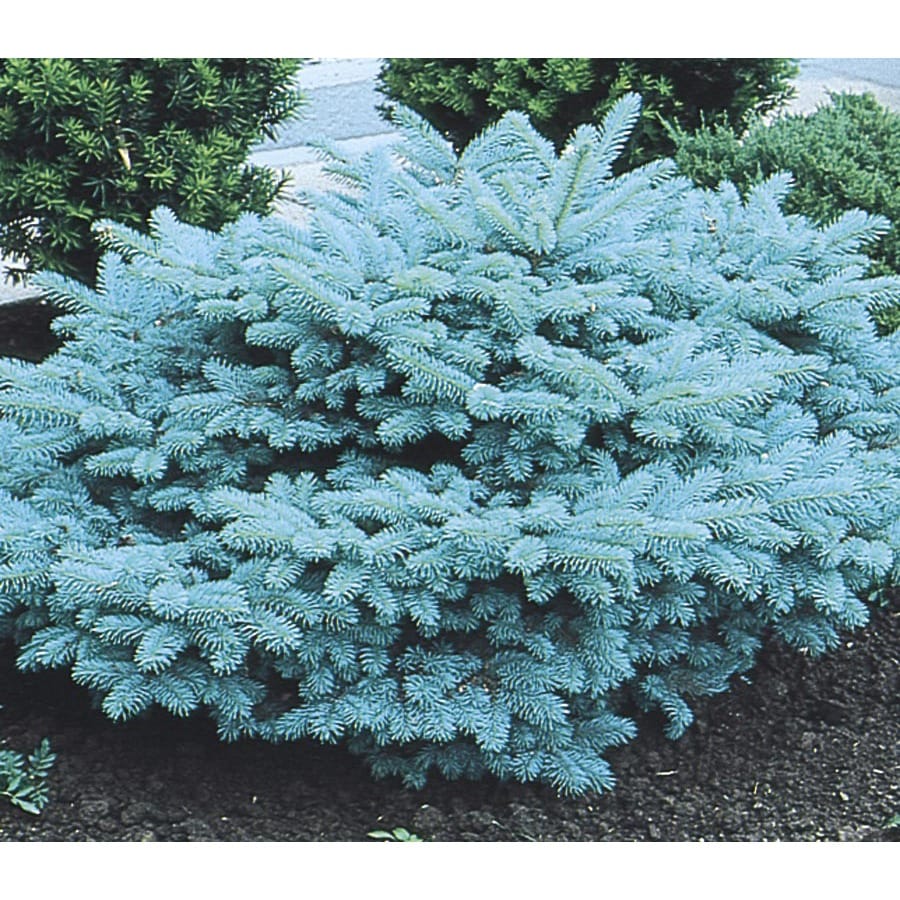This horizontal rectangular image predominantly features a unique light bluish-green evergreen bush, filling most of the center. The bush, which has a striking blue or aqua hue, sits in the foreground with dark soil or mulch at its base. In the background, dark green evergreen bushes are visible, hinting at their larger size. The upper left corner shows a patch of sky and some clouds, but the center-left background seems to reveal the side of a house, potentially indicating a residential setting common in the Midwest or East. Beyond the darker green shrubs, pavement is present, suggesting nearby sidewalk or street access. The image is taken during daytime, evident from the clear and well-lit surroundings.